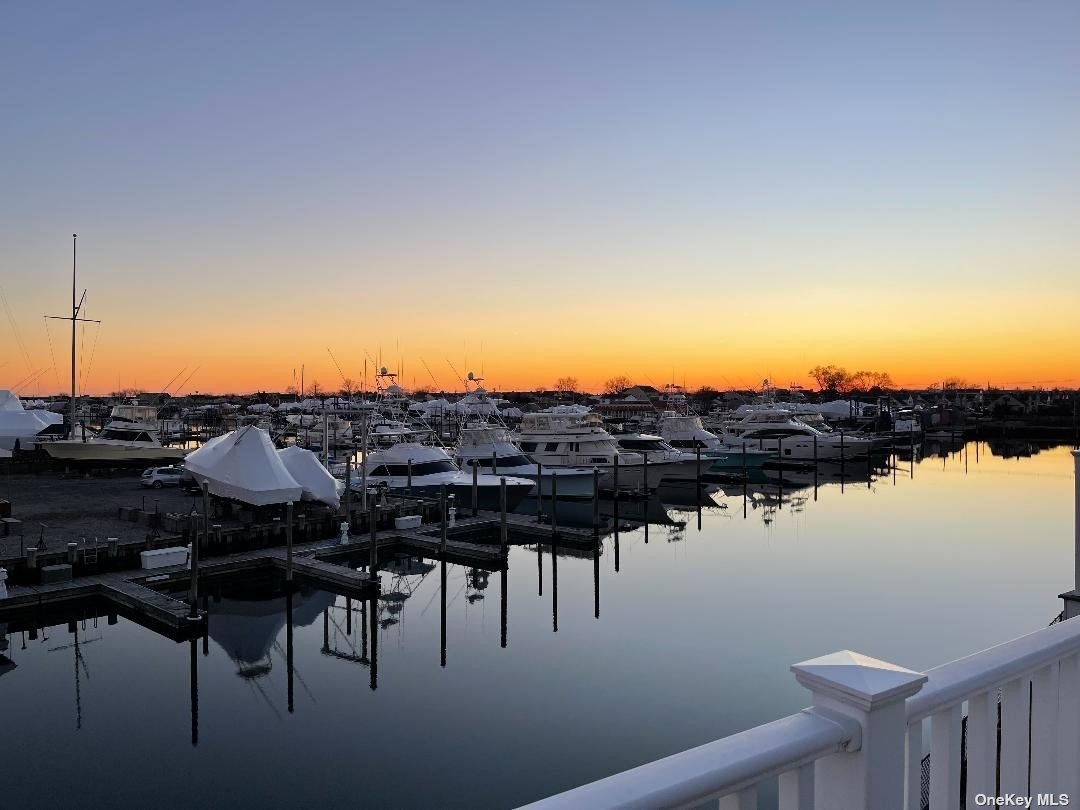The photograph captures a tranquil marina scene just past sunset or possibly at the break of dawn. The image, seemingly taken from a balcony or porch of a nearby building, includes a white plastic railing in the foreground. Beyond this barrier lies the serene waterway, with numerous white yachts and boats docked at the harbor. The horizon is framed by leafless tree silhouettes, creating a stark contrast against the vibrant gradient of the sky, which transitions from a deep blue at the top to rich yellow and orange hues closer to the horizon. Shadows cast by the boats elongate across the still water, enhancing the calm atmosphere. The image is accented with the text "One Key MLS" in the corner, indicating a possible real estate listing or branding.